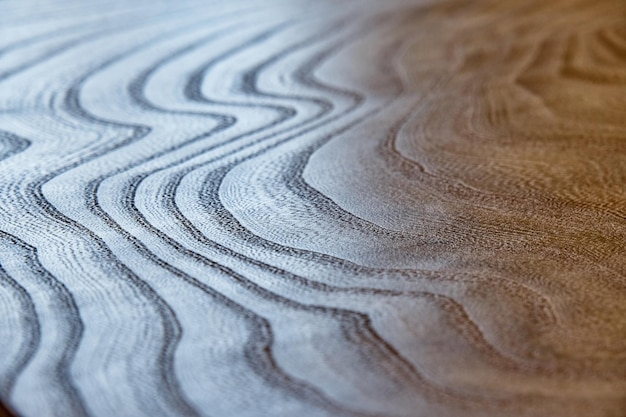The image captures a textured surface that evokes the natural grain patterns of wood or the wavy designs of sandy soil. The surface predominantly features shades of gray, with the left portion appearing light gray due to the way light hits it, and the right part exhibiting a reddish-brown hue, possibly because of different lighting, such as sunlight or a sunset. The surface is marked by undulating lines that extend from top to bottom and create a repeating pattern, though these lines are more defined on the left two-thirds of the image, becoming less distinct on the right. The photograph appears to be taken at an angle, focusing intently on this intricate, wavy texture, leaving the setting—whether indoors or outdoors—ambiguous.